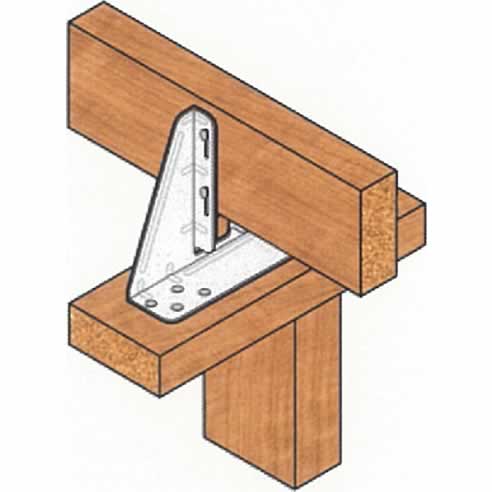The hand-drawn and hand-colored image depicts a detailed diagram of a joint connecting three wooden planks, arranged to illustrate a specific structural setup. The drawing portrays one vertical rectangular plank standing upright from bottom to top. Perpendicular to this upright plank, an horizontal plank intersects it mid-height, resembling the top of the letter 'T'. Secured to the intersection is an L-shaped metal bracket with a total of six holes — four in the horizontal section attached to the T-top plank and two in the triangular extension of the bracket which affixes to the third plank that lies on top of the T-joint. This third plank is slanted and highlights how the bracket holds and aligns all three pieces of wood together. The background is a solid off-white, creating a stark contrast that makes the planks, colored in varying shades of brown with black edges, and the white bracket appear to float in a white void. The positioning and detailed nature of the illustration suggest it may serve as a clearer instructional tool, perhaps used in a woodshop to show precise construction or assembly techniques.